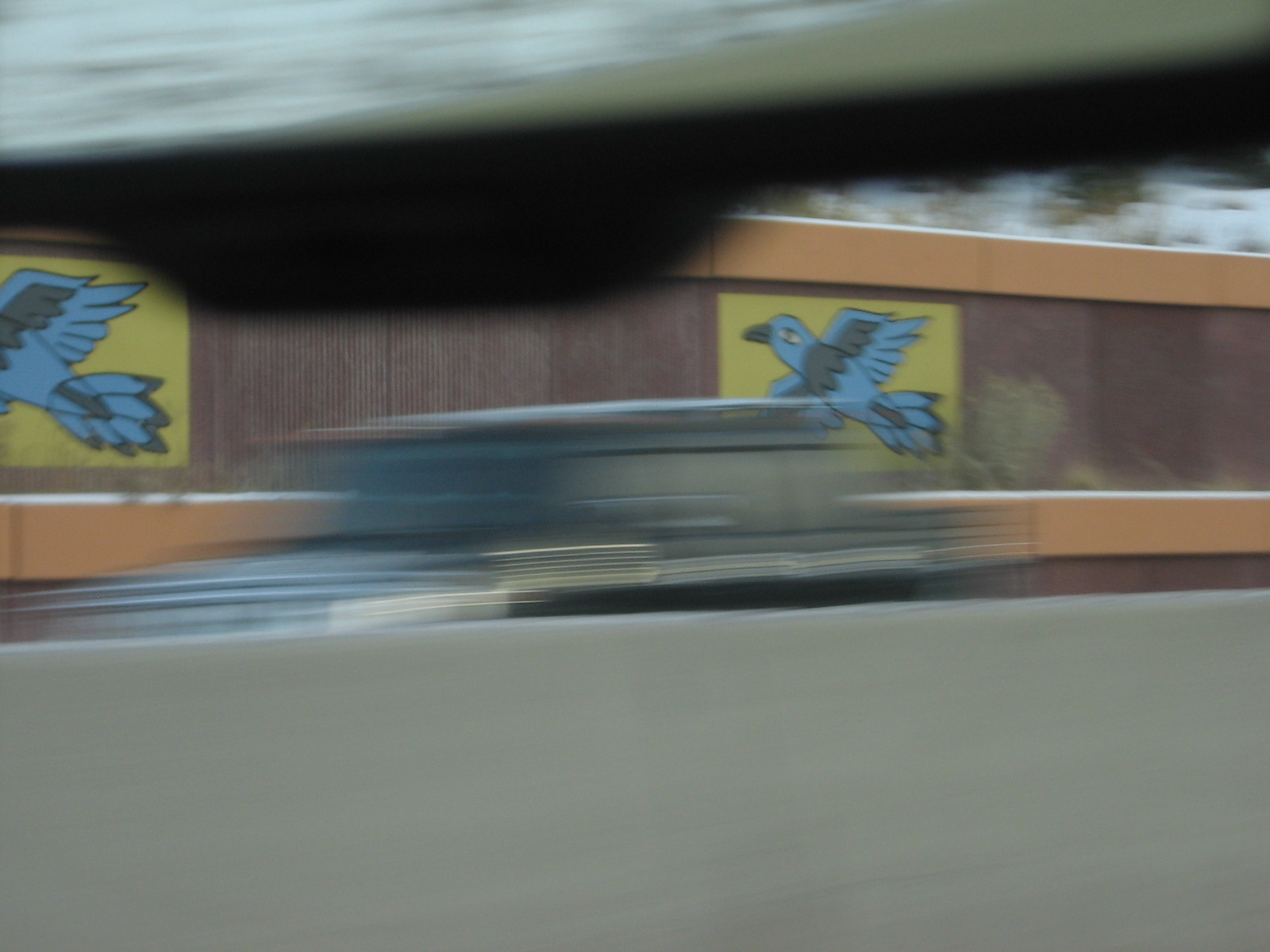In this image, a blurred close-up reveals a scene that is somewhat difficult to discern. At the top, there is a horizontal gray line that appears to be part of an obstruction through which the photo is taken. Beneath this gray line is a thin black line, adding to the visual segmentation. In the background, there is a slightly blurry indication of an outdoor scene that includes a faint glimpse of a blue sky and some indistinct trees. A fence is also visible, characterized by a tan top rail and vertical wooden slats with a faux grain pattern.

Within this scene, two distinct tiles or squares are present. They are gold in color and feature a blue bird in flight. One tile is located slightly to the right of the image's center, while the second one is partially visible on the left. Between these two bird-decorated tiles, three wooden slats are visible, making the bird on the second tile partially obscured. Below these tiles is another light tan bar, paralleling the one at the top of the fence. The entire image is viewed through a grayish, partially obstructing object, adding a layer of visual complexity to the scene.